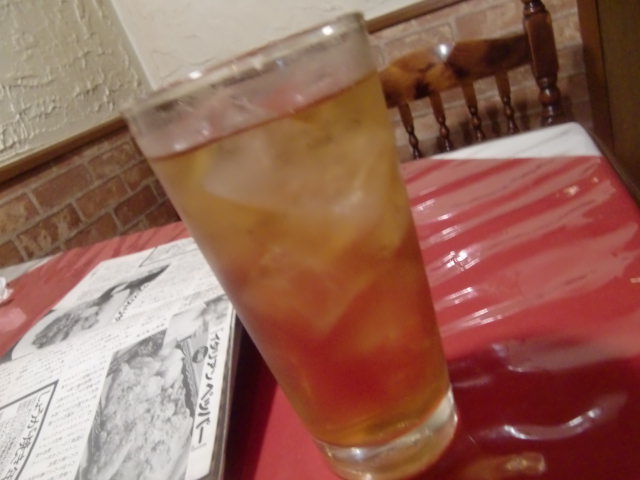This close-up image captures a glass filled with a light brown liquid, likely iced tea, with several ice cubes floating in it. The glass, which appears to be a 16-ounce pint size, is set on a table covered with a red tablecloth that has a clear plastic overlay. To the left of the glass, there is a black-and-white menu booklet featuring bars of black text and grayscale photos, and what appears to be some writing in an Asian language. In the background, you can see a dark woodgrain chair with intricately turned spindles, positioned in front of a textured white stucco wall with a brick pattern on the lower half. The table is placed in a corner of the room, adding to the cozy, slightly blurry ambiance of what seems to be a restaurant setting.